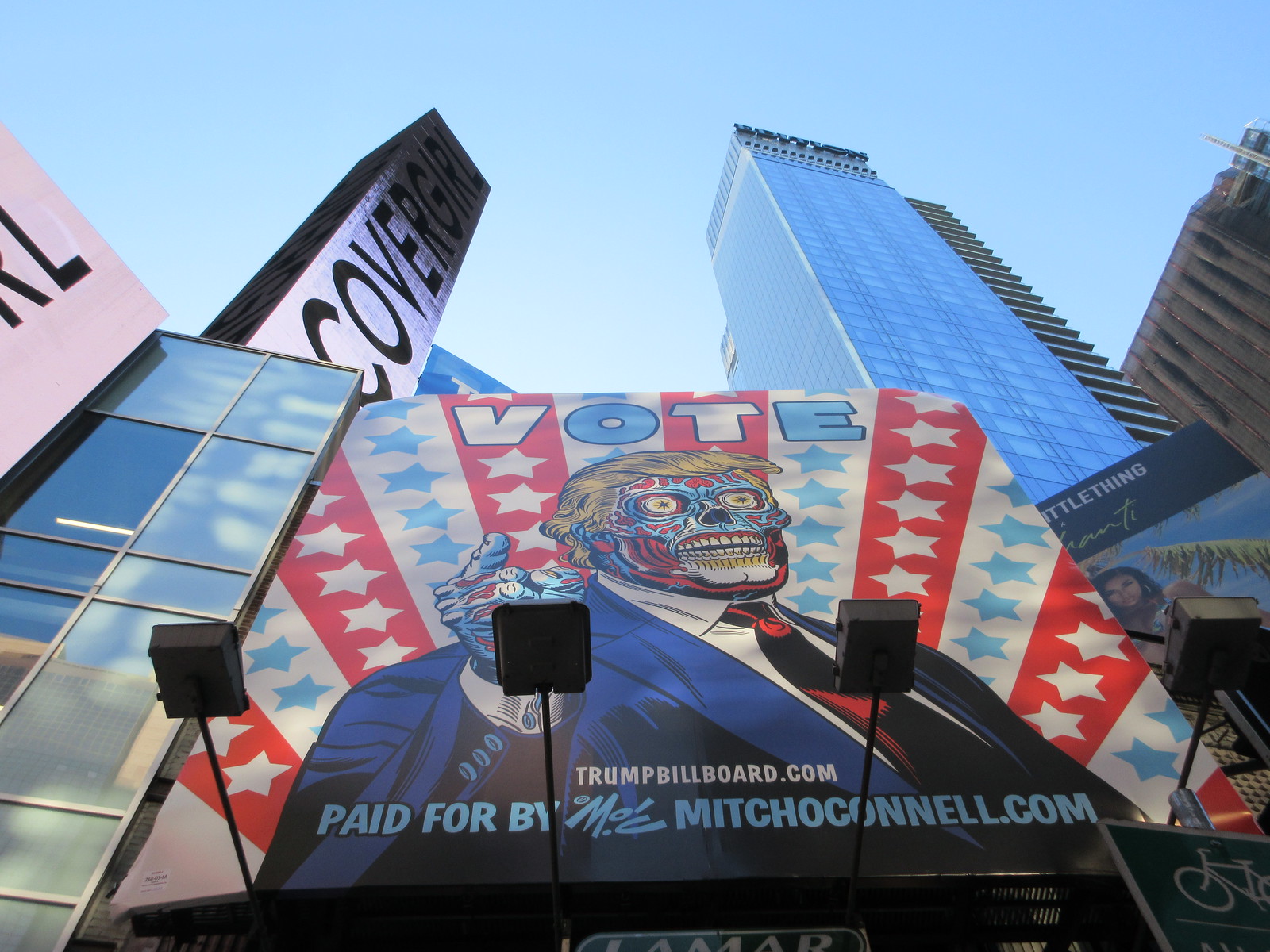In this photograph, set in the bustling downtown area, several towering skyscrapers punctuate the skyline. Among these buildings, the leftmost skyscraper prominently displays the name "Covergirl" on its purplish facade, juxtaposed beside a pink building and others adorned with reflective windows. On the right side of the image, a brown building stands out.

Dominating the scene is a satirical and striking billboard featuring a grotesque parody of Donald Trump. His skin appears peeled away, revealing exposed muscle and bone, while a blue hue tints his face. Trump's eyes are bloodshot and reddened, his teeth twisted into a snarl, yet his iconic blonde hair remains unmistakable.

The background of the billboard showcases vivid red, white, and blue stars and stripes, and at the bottom, the websites "trumpbillboard.com" and "moemitchmcconnell.com" are noted in white text. Trump is depicted wearing his characteristic dark blue suit, complemented by a long red tie and a white shirt. The billboard, paid for by the aforementioned website, adds a layer of dark satire to the urban landscape.